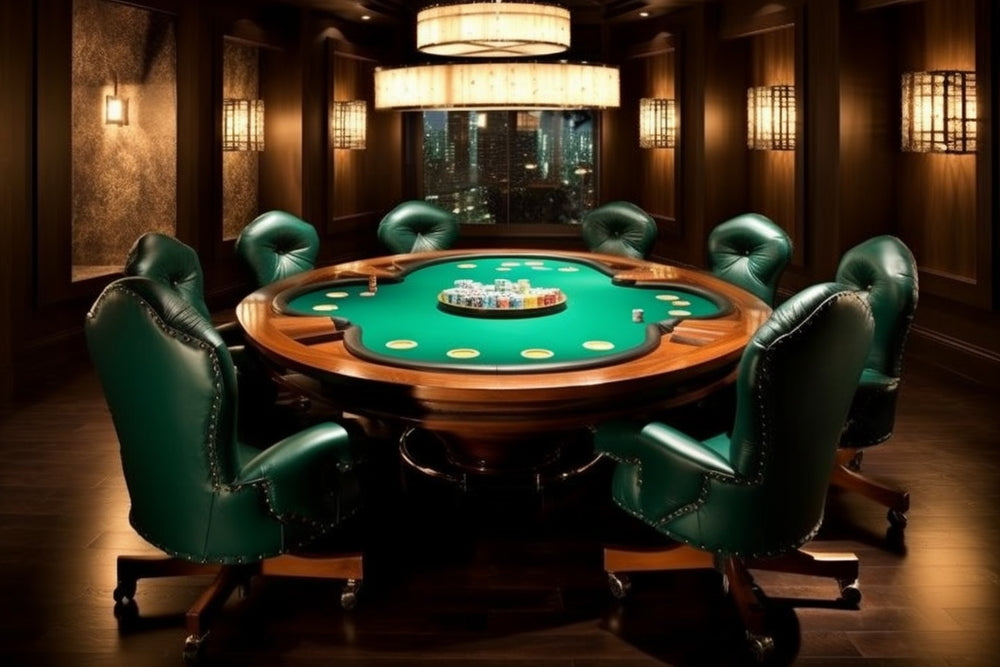The image captures an elegant indoor space centered around a luxurious poker table with a green felt top and a polished wooden edge. The table, which has a circular design, includes features like numerous cup holders and a padded black material surrounding the felt. The middle of the table is cluttered with poker chips in various colors—reds, greens, blues, and whites—alongside plastic coins and dice. Surrounding the table are eight high-back, plush green leather chairs, each adorned with rivets and equipped with wooden legs ending in small wheels, suggesting a blend of opulence and functionality.

The room itself is richly detailed, with dark wooden walls that have lighter brown trim and sections housing brown box-like lanterns which emit a soft white light. A prominent chandelier hangs from the ceiling, casting a bright illumination over the table. Additionally, there is a window providing a view that hints at a cityscape beyond, visible through the specks of light that mimic city lights. The floor is made of dark brown tiles, further adding to the room’s sophisticated ambiance.